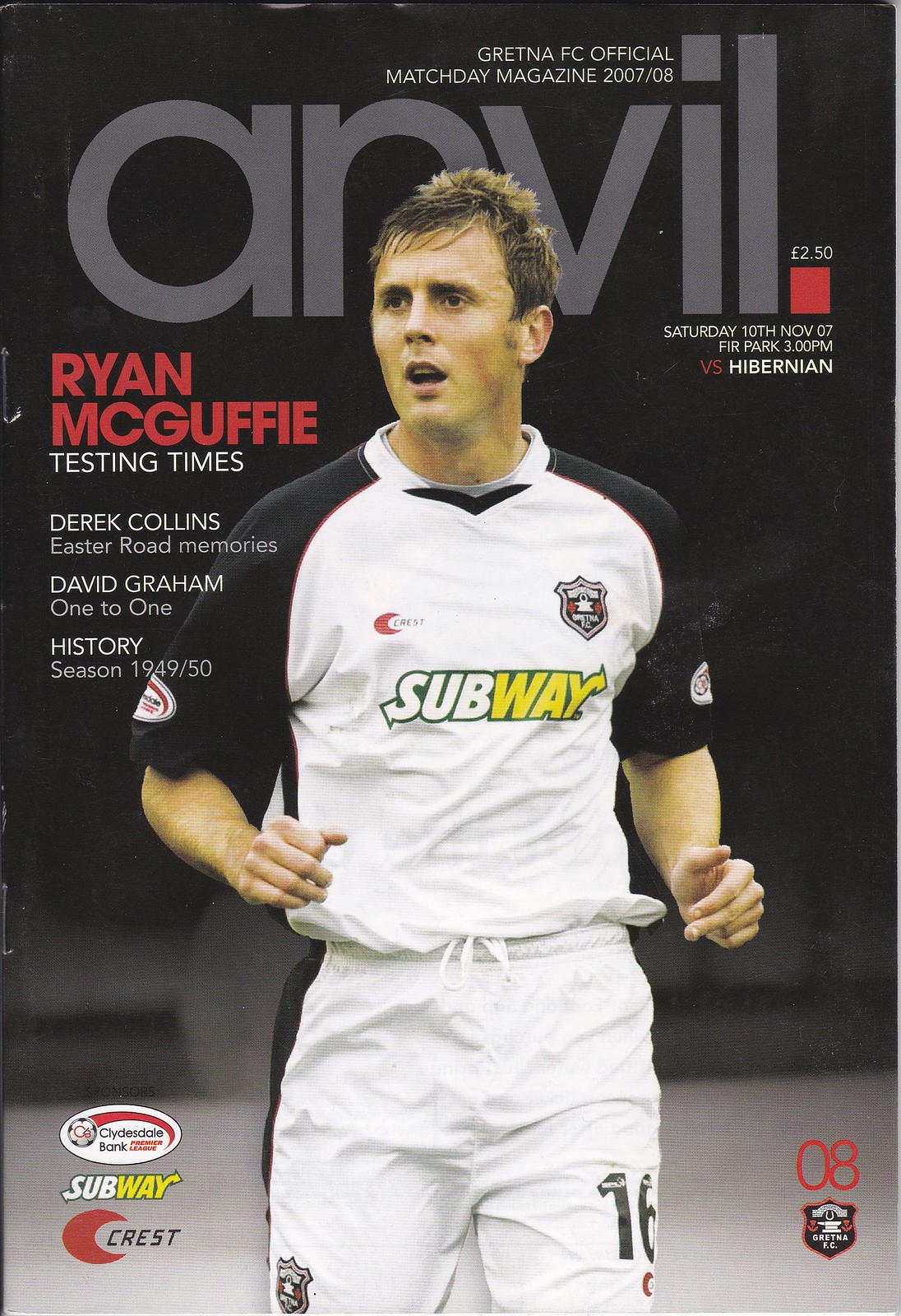The cover of Anvil Magazine features an action shot of athlete Ryan McGuffey mid-run on a soccer field, wearing a black-and-white jersey with the iconic Subway logo prominently displayed across the chest. His team logo is positioned on the upper left of his shirt, complemented by white pants. McGuffey's name is highlighted in red on the right side of the cover, alongside the title of the main article about him, "Testing Times.” The magazine, priced at 2.5 euros, also announces other articles such as "Derek Collins: Easter Road Memories" and "David Graham: 1-1, History Season, 1949-50." This edition, released for Match Day on Saturday, November 10, 2007, against Hibernian, prominently displays the logos of Subway and Crest at the bottom. The backdrop of the cover is black with the magazine title "Anvil" in gray at the top, and features the colors black, white, gray, yellow, green, and red throughout. This cover serves as the official magazine of Gretna FC for the 2007-08 season.